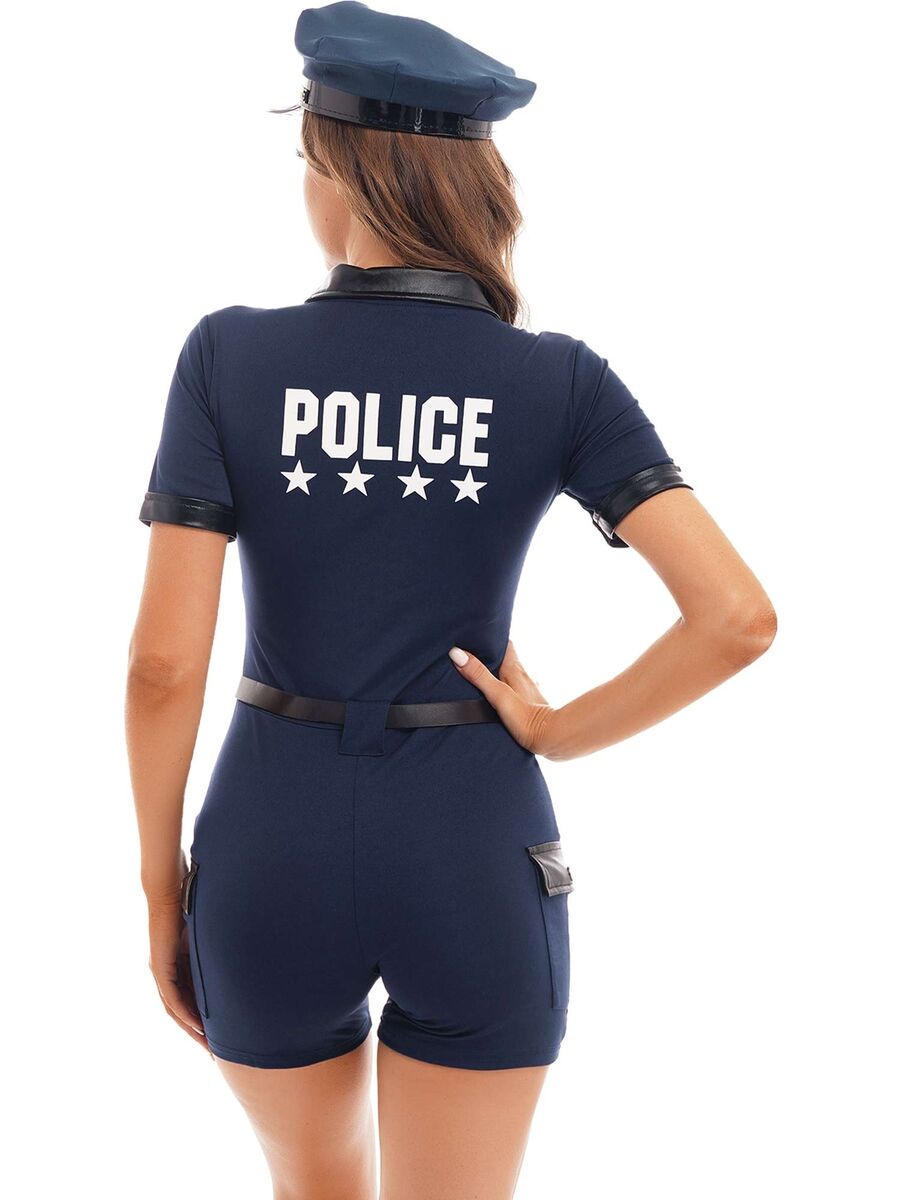This image, set against a plain white background, features what appears to be a woman or possibly a realistic doll. It is difficult to determine the exact nature of the figure due to the smooth and shiny quality of the light-colored skin, which suggests either a high degree of photo editing or a hyper-realistic rendering. The subject is viewed from behind, from the knees up to the top of the head, with a slight turn to the front left that reveals a hint of her cheek but not her face.

The woman, seemingly in her 20s or 30s, has long, reddish-brown hair swept over her right shoulder. She is dressed in a blue costume resembling a police uniform, complete with short sleeves and short pants. Her uniform features distinctive details: "POLICE" is printed in bold white letters across the back, accompanied by four evenly spaced white stars. The outfit includes a black leather thin belt, black bands around the sleeves, and black leather flaps on the pockets of her shorts. Additionally, the collar of the shirt also has black leather accents.

Completing the look is a navy police cap with a black leather band matching the rest of the outfit. The woman’s right hand is placed on her right hip, showcasing white fingernails. The overall ensemble, with its numerous leather details and the slightly exaggerated features, suggests that it might be more of a costume rather than an authentic police uniform.